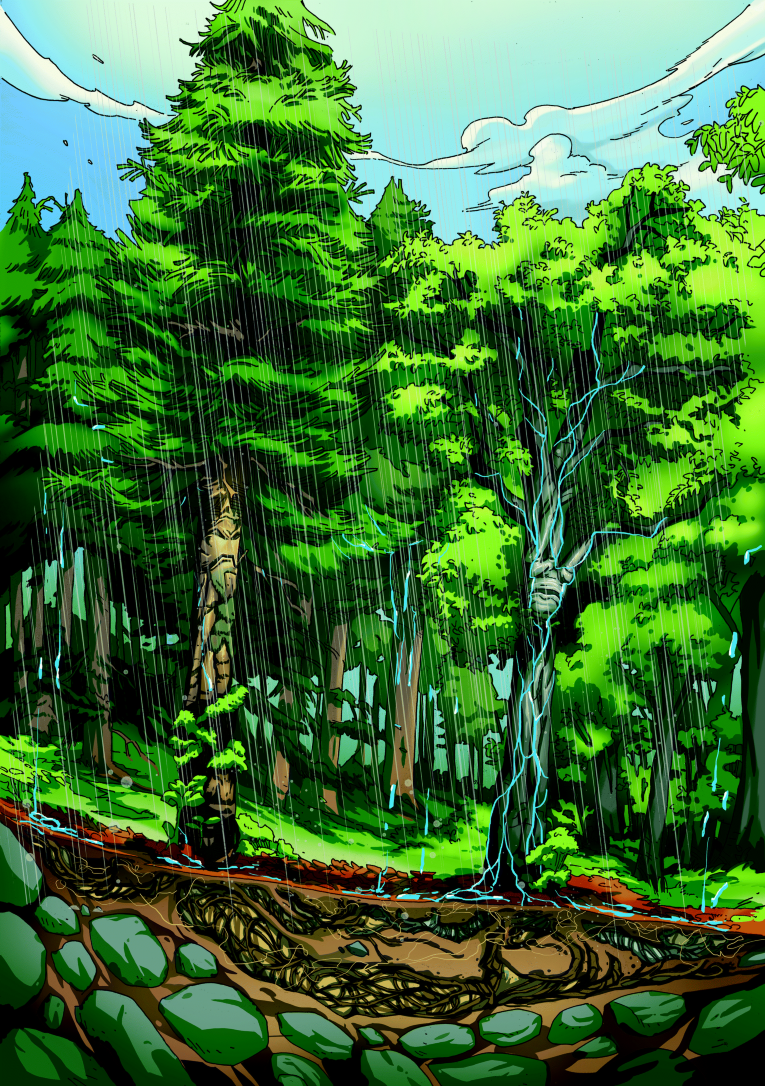The digital image, reminiscent of a cartoon or comic book, is vertically aligned and vividly captures a rainy outdoor forest scene. The sky at the top is depicted with a blend of light yellow and blue hues, transitioning into white clouds outlined in black pen strokes. Diagonal gray lines densely fill the sky, representing the falling rain. Dominating the middle section are tall pine and cedar trees, characterized by their brown trunks and green foliage. Interestingly, some trunks feature faces, adding a whimsical touch; the taller trees on the left display stern expressions while the bushier trees on the right exhibit fearful or angry faces, and their trunks appear blue-gray.

Beneath the forest floor, the brown dirt is visible, showcasing the extensive root systems of the trees. One central tree prominently features blue-highlighted roots, resembling bolts of lightning. At the very bottom of the image, irregularly shaped green rocks are embedded within the soil, completing this multi-layered, detailed depiction of a natural scene interlaced with fantastical elements.